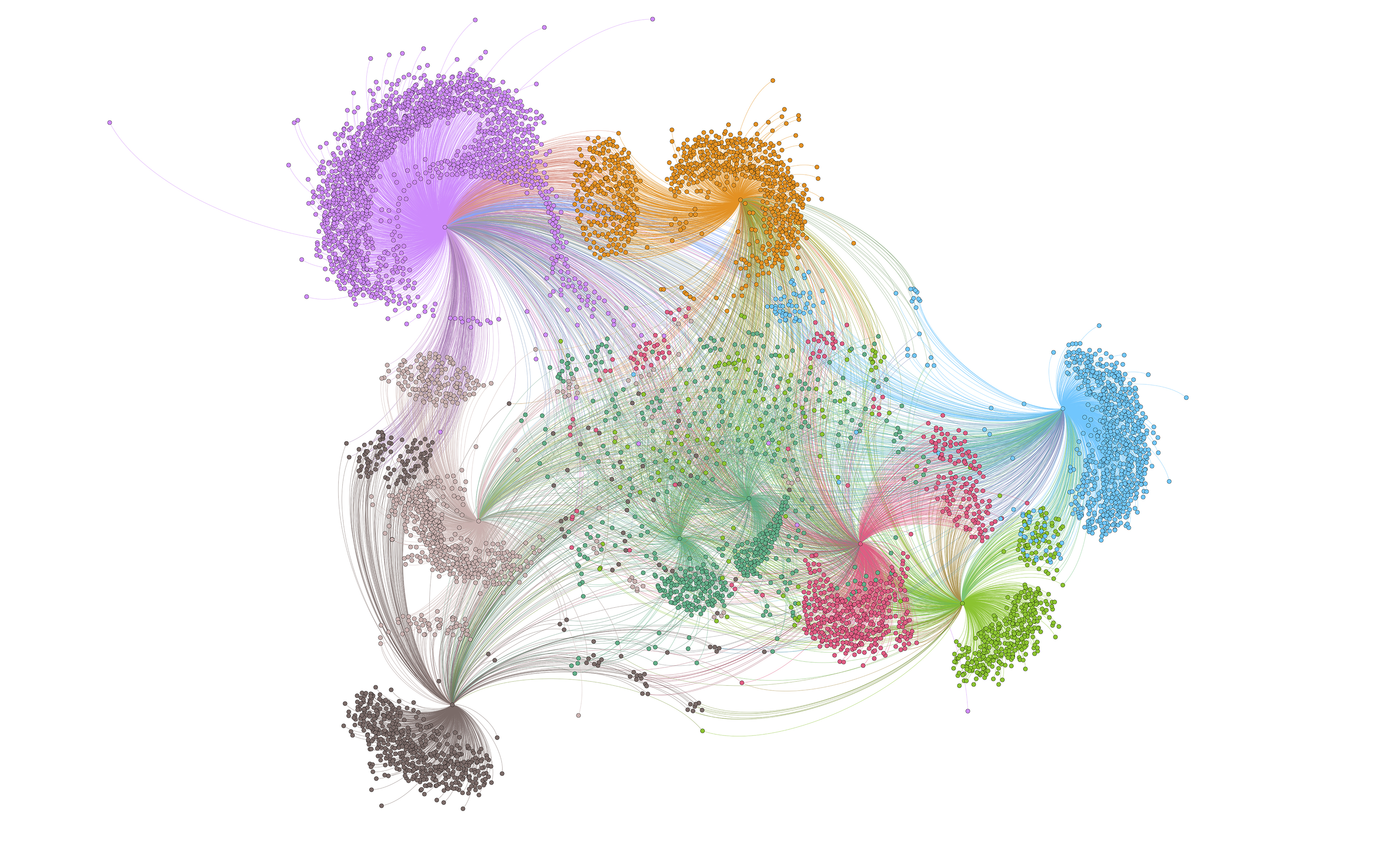The image displays an intricate and vibrant abstract ink drawing resembling a whimsical collection of multicolored dandelion seed tops interconnected by a myriad of fine, swirling lines. The composition cascades with a variety of hues, starting with a vibrant purple section in the upper left, followed by two deep burnt orange areas towards the middle. In the far right center, a beautiful shade of baby blue contrasts against a lush green placed directly below it. Surrounding this green, there is a playful scattering of lime green, dark pink, and a striking vibrant red with encapsulating bursts of dots. A dark green sits prominently in the middle, creating a central anchor point for the composition, alongside a gray rendition to the left of it and a monochromatic black one towards the bottom. The entire scene forms an expansive and dynamic display, with the lines and dots evoking a sense of fluid movement and interconnectedness, ultimately giving the impression of seeds or particles exploding into a radiant kaleidoscope of colors.